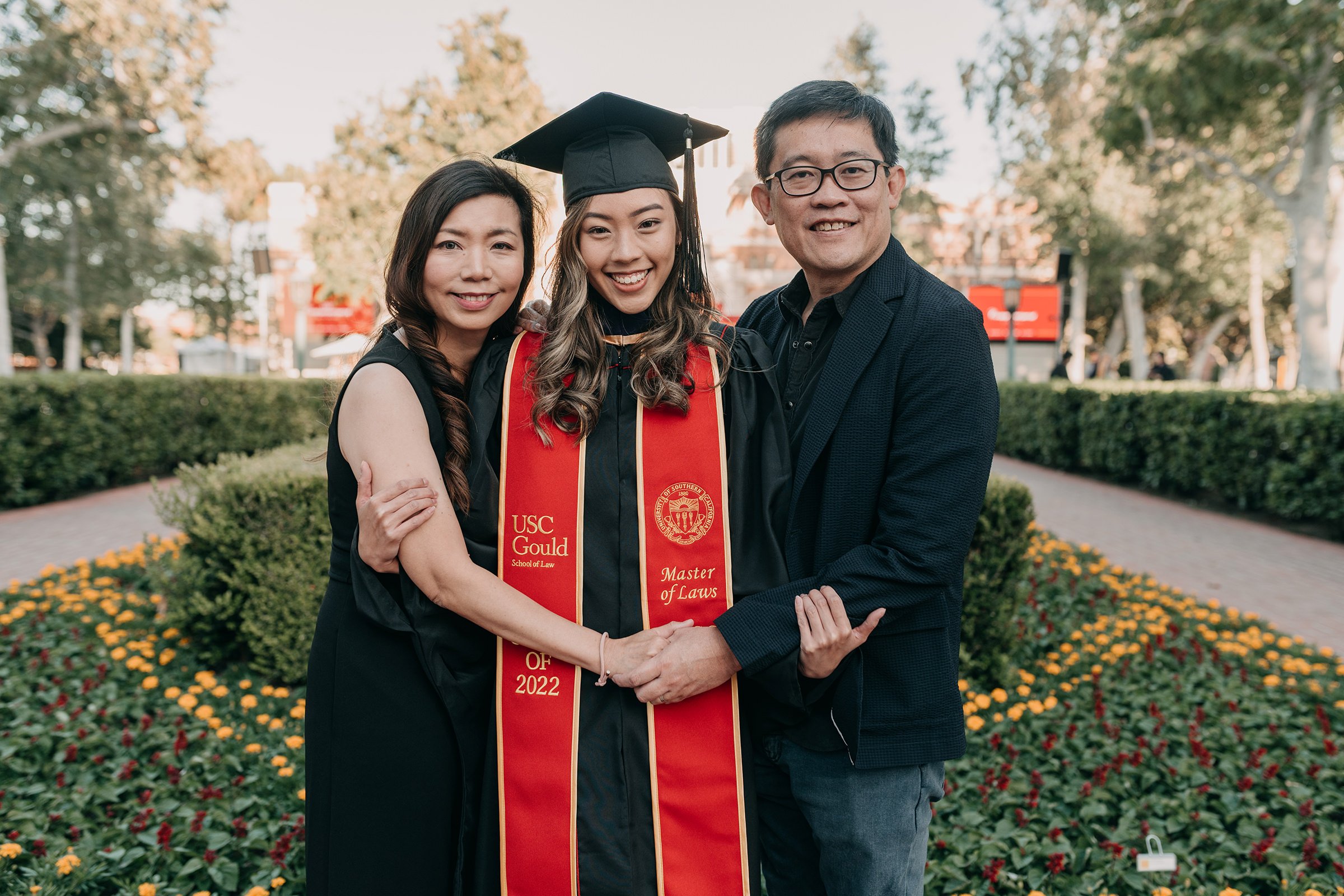In the foreground of this detailed image, a proud Asian family—comprised of a mother, father, and daughter—stands together to celebrate the daughter's graduation. The father, positioned on the right, has short black hair, wears black-framed glasses, and is smiling. He is dressed in a black sport coat, black long-sleeve business shirt, and blue denim Levi-type jeans. The mother, with styled long black hair cascading to her mid-shoulders, is elegantly dressed in a black dress. At the center, the beaming daughter wears a black graduation cap with a black tassel, and a matching black gown adorned with a red sash bordered in gold. The sash proudly announces “USC Gould, Master of Laws, Class of 2022.” The family stands in front of a neatly manicured flower bed that forms a V on both sides, bounded by low, straight groomed hedges and adjacent sidewalks. In the background, there are trees and a red building, complementing the vibrant scene of this significant milestone.